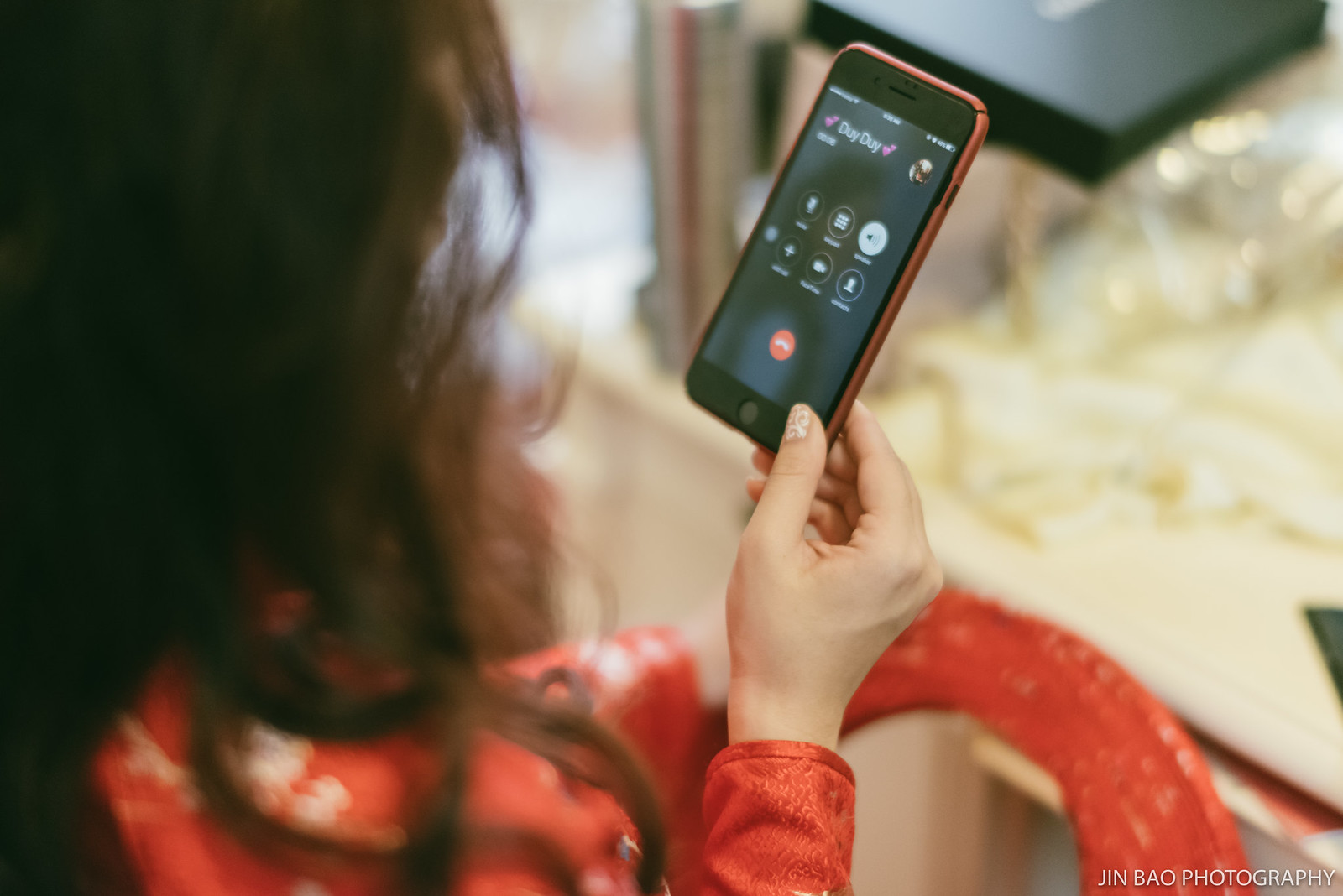The photograph captures a woman with long, dark brown hair, dressed in a red long-sleeved dress or blouse. She is indoors, and the image is rectangular, wider than it is tall, mostly focusing on her and the cell phone she holds in her right hand. The left side of the frame prominently features her hair against a black backdrop. The woman, who appears to have pale skin and finely manicured nails with a tan background and white swirl design, is looking at her cell phone. The phone she holds has a ruby red cover, and its screen displays the text "DUI DUI" outlined in hearts, along with various app buttons. The screen also shows "00:08," suggesting she is on a phone call. The background on the right half of the picture is blurred to keep the focus on the phone and her hand. Below her, the surface appears to be a light tan table or countertop, potentially with a black box and some see-through plastic packaging on it.